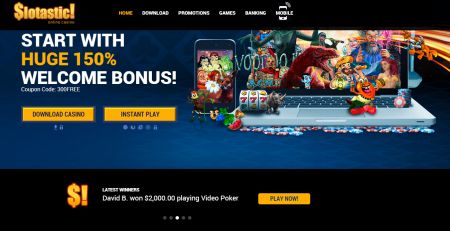The image depicts a computer screen displaying the homepage of a website with a predominantly black background. In the upper left corner, the logo "Slotastic" is featured with a stylized dollar sign replacing the 'S.' To the right of the logo, there are navigation options including "Home," "Games," and "Banking," with the homepage currently selected.

Central to the screen is an image of an open laptop displaying various games. One game showcases a wheel with three number sevens, a symbol often associated with winning in slot games. Other visual elements include a princess with yellow hair and a small, fuzzy red character.

On the left side of the screen, white text reads, "Start with," followed by "huge 150%" in yellow, and "welcome bonus" in white. Below this text, there are two yellow buttons labeled "Download Casino" on the left and "Instant Play" on the right.

At the bottom of the screen, there's an announcement featuring a dollar sign and an exclamation mark, stating, "David B won $2,000 playing video poker." Adjacent to this, a yellow "Play Now" button is displayed.